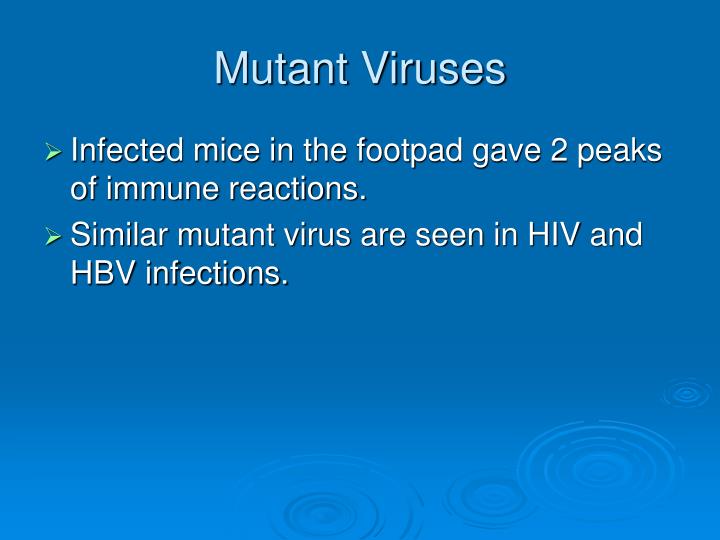The image is a PowerPoint slide with a blue background featuring subtle water droplet rings at the lower right corner. Centered at the top in white Arial font is the title "Mutant Viruses." Below the title are two bullet points, each marked with right-facing green arrows. The first bullet point reads, "Infected mice in the foot pad gave two peaks of immune reactions." The second states, "Similar mutant virus are seen in HIV and HBV infections." The text is white, and the layout is clean with no additional images or elements other than the blue background and water ring effects.